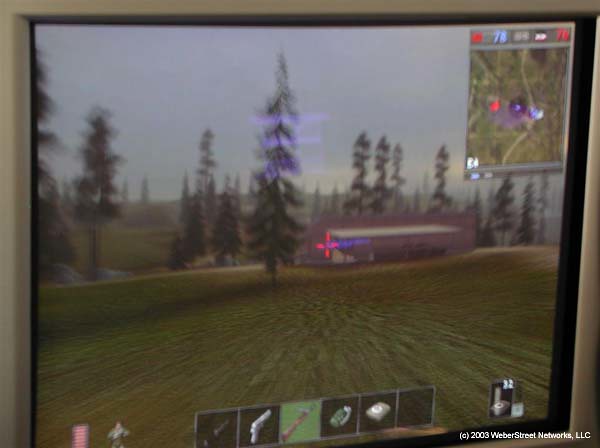This image captures a scene from an old-school, pixelated video game displayed on a computer monitor with a silver or gray border. The game appears to be a first-person shooter with survival elements, as indicated by the assortment of tools and weapons, including a silver pistol, a brown rifle, a green grenade, a green bandage kit, and an axe with a black handle shown in the bottom center inventory. The gameplay interface includes a reticule at the center screen, health status, ammunition count, and a possible currency indicator on the right. An overhead map is visible in the top right corner, showing the character's location and other notable spots. The scene within the game is set in an open grassy field with tall green pine trees, resembling a forest area, and features a large brown building that the character appears to be approaching. The monitor’s bottom right corner displays a copyright notice: "2003 Weber Street Networks, LLC."